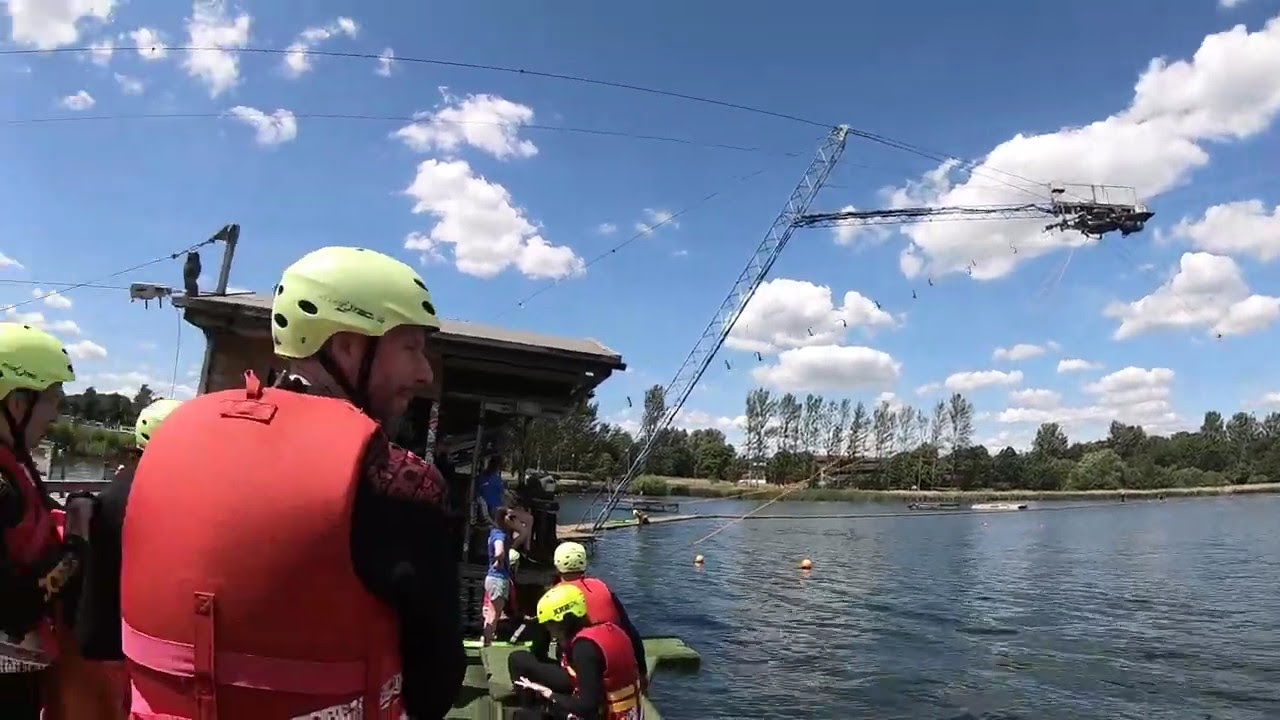In this vivid landscape-oriented color photograph, we see a dynamic waterside scene of either a lake or a river. The image is dominated by a brilliant blue sky filled with fluffy white clouds, which takes up the top two-thirds of the frame. The dark blue water, sunlit on the right lower part of the image, contrasts beautifully with the shoreline on the left. This shore is bustling with activity as several men, all wearing fluorescent yellow helmets and orangish-red life jackets, gather around a partially open, roofed structure. This structure seems to be associated with some filming activity, as suggested by a boom or crane arm extending diagonally into the sky from the rear of the structure, and cables dangle from it pointing towards the water. The far bank of the lake is lined with a dense row of trees, adding a serene natural backdrop to the scene. In the foreground, some participants are seen seated, all facing away from the viewer and towards the water, contributing to a sense of anticipation and teamwork. Overall, the photograph captures a crisp, realistic moment of what appears to be an organized and potentially technical outdoor activity beside the tranquil but engaging waterscape.